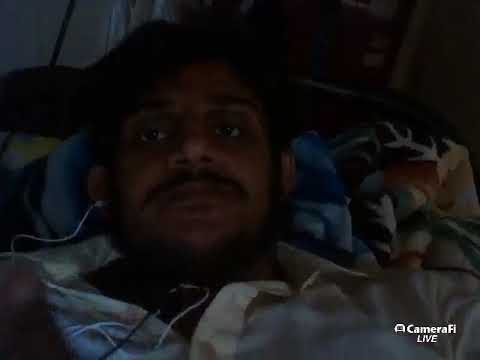In this detailed photograph, a man of possibly Indian or Middle Eastern descent, likely in his 30s or 40s, is depicted from his upper chest to the top of his head, laying back on what appears to be a bed. His attire consists of a blue and white polo shirt with the collar buttons undone. The man is outfitted with a single earbud in his right ear, connected by a white wire that runs downward, partially visible against his chest. His facial features include a mustache, a patchy beard, dark eyes, and black hair brushed to the left. Behind him, a variety of soft blankets in different styles and colors, including blue and black-and-white, create a textured backdrop. The image has a somewhat dark and shadowy ambiance, making finer details harder to discern. In the bottom right corner, there is white text that reads "CameraFi Live," with "CameraFi" capitalized as C-A-M-E-R-A-F-I and "LIVE" in all uppercase letters, suggesting the use of a third-party camera application. The man gazes at the camera without a smile, displaying a neutral expression.